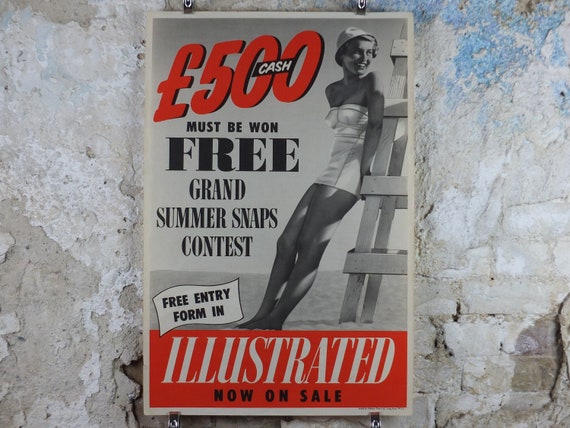This image is a photograph of an old magazine poster mounted on a rough brick wall, featuring a combination of exposed brickwork and weathered plaster. The bricks are a mix of dark and light gray, with spotted blue paint in the upper right corner, and are most defined in the lower right section. The vertical rectangular poster is affixed to the wall with silver clamps. 

The poster itself showcases a black and white photograph of a young woman at the beach, leaning against a white lifeguard tower positioned to the right. She is wearing a retro-style strapless white bathing suit that covers her chest and extends down to her buttocks, along with a white bucket hat over her short blonde hair. She stands on the sand, smiling and gazing off into the distance towards the right.

The text on the poster is a vibrant combination with striking details. At the top, it reads "£500 euros cash" in bright red font, with the word "cash" enclosed in a black box with white font. Below that, in a black font, it states, "must be won - free Grand Summer Snaps contest." Further down, "free entry form in" is written in black text within a white flag that has a black border. At the bottom, a red banner features the phrase "Illustrated, now on sale," with "illustrated" in white italicized font and "now on sale" in black font.